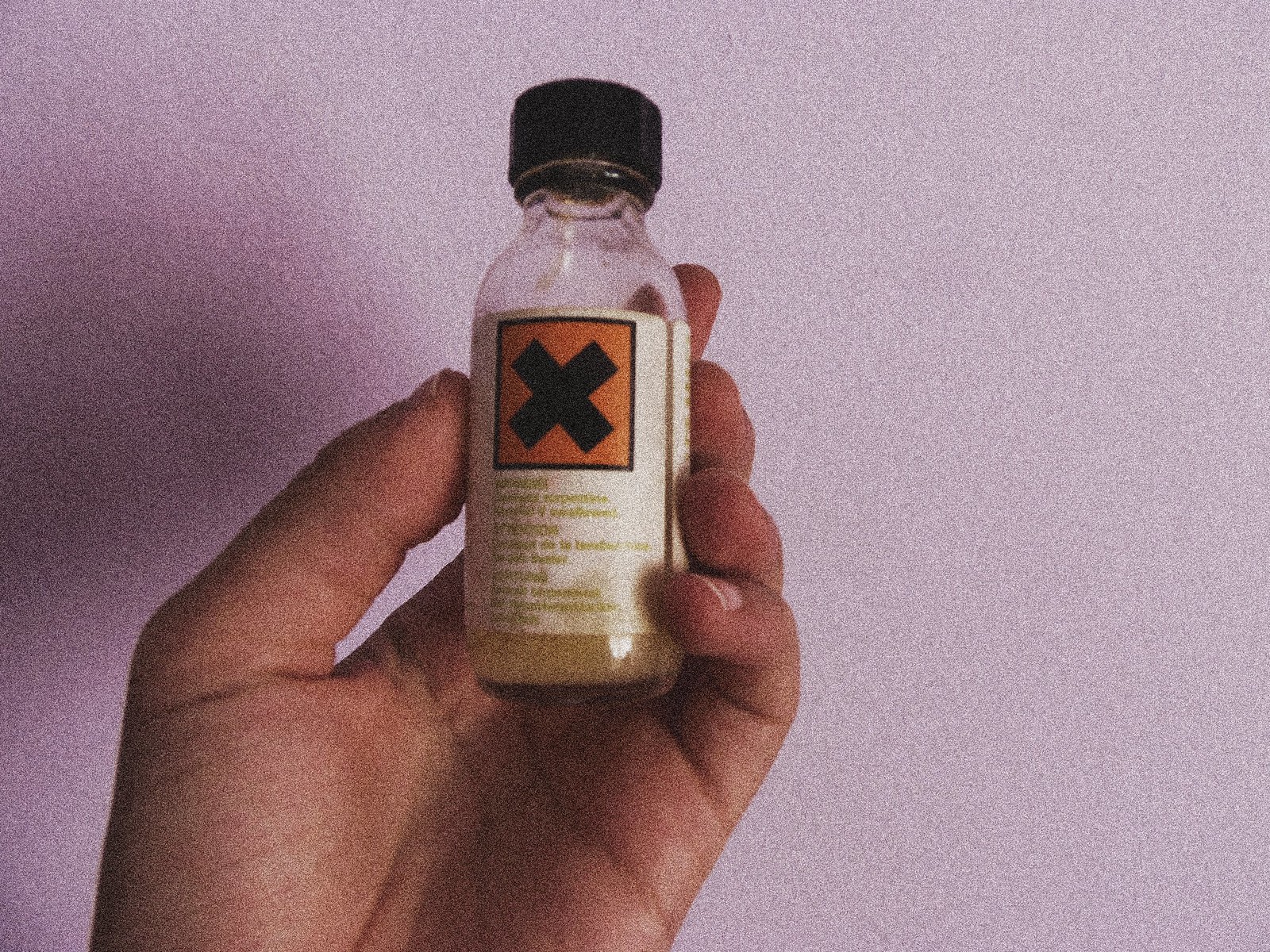In the image, a Caucasian hand with nicely trimmed, manicured nails is holding a small, clear medicine vial. The bottle has a tight black cap and contains a brownish liquid, akin to the color of burnt butter, with only a small amount left inside. The label on the bottle features a prominent orange square with a bold black X in the center, accompanied by some unreadable text due to the blurriness. The background is a grey wall, casting a shadow from the hand, and the overall setting suggests either a laboratory environment or a personal apartment. The image highlights the mysterious and potentially hazardous nature of the vial, conjuring caution due to the ominous labeling.